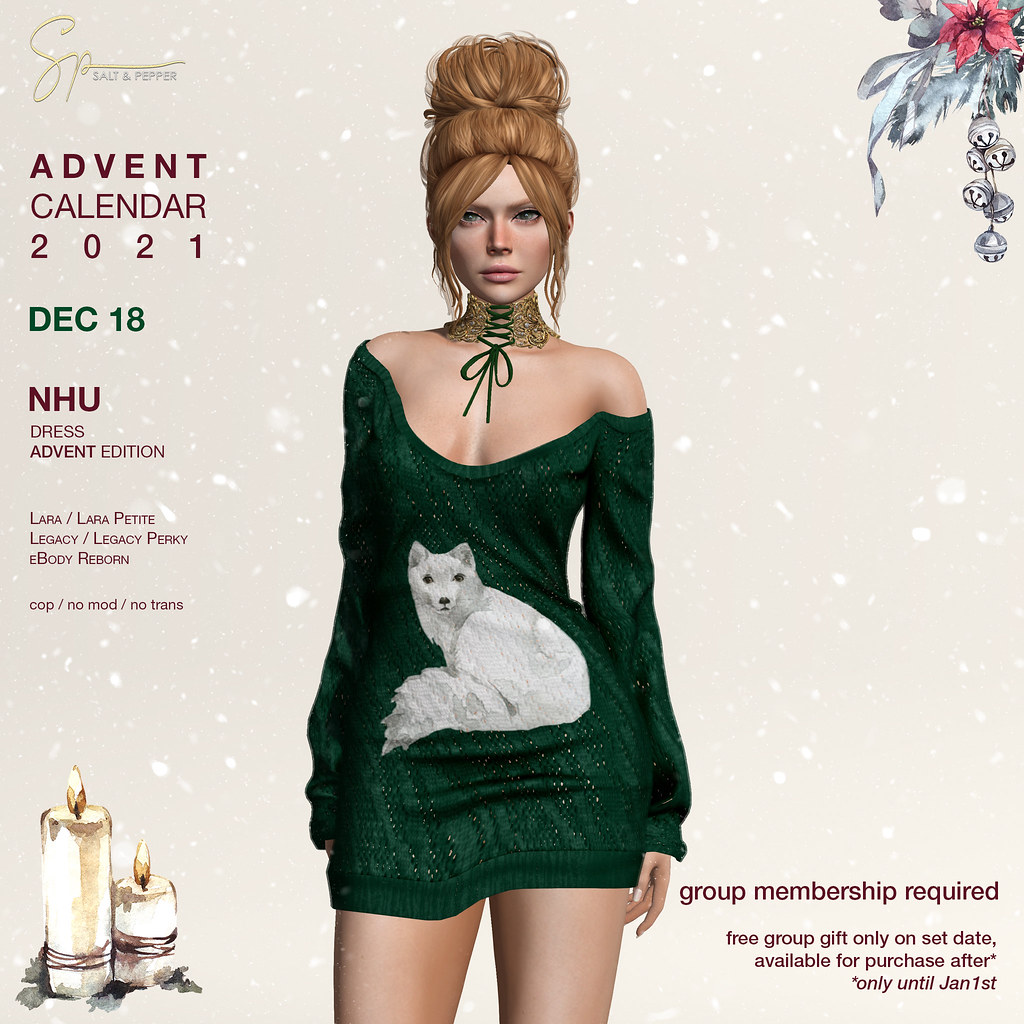The image is an advertisement flyer for a December holiday event showcasing a 3D-rendered, video game-like woman. She has reddish-auburn hair styled in an elegant double bun, with a golden collar adorned with a green ribbon around her neck. She dons a striking green dress that doubles as a mini-skirt, featuring a prominent painting of a white wolf. Her facial expression exudes confidence. In the top left corner of the flyer, it says "Salt and Pepper" and "Advent Calendar 2021, December 18th, NHU Dress Advent Edition," alongside names such as Laura Petit, Legacy Perky, and eBody Reborn, indicating compatibility or sponsorship. Additional text notes "Cop, No Mod, No Trans." Decorative elements include a pink flower and white Christmas bells at the top right, burning animated candles at the bottom left, and snow in the background. The bottom right details that group membership is required for a free group gift available only on the set date, purchasable after only until January 1st.